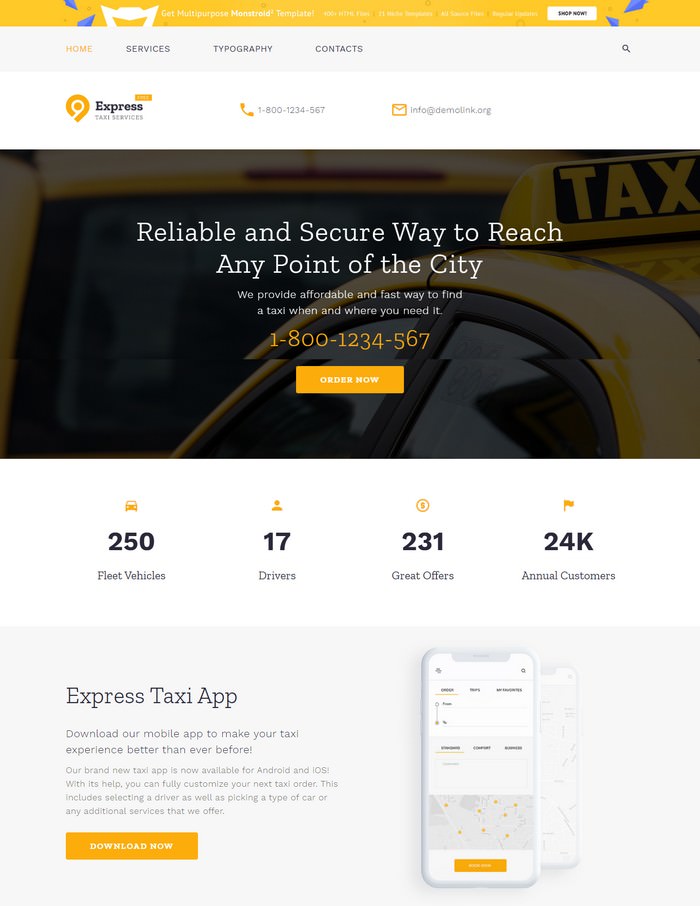The image showcases the ExpressTaxi app interface, featuring a user-friendly design with a prominent yellow header that clearly displays the app's name. Central to the header is a distinctive yellow pin icon, reminiscent of a map pin with a unique form that does not connect at the bottom. The main interface provides options for contacting customer support via an 800 number and a .org email address.

The app offers several navigation choices including "Photography," "Contacts," and "Home." Below these options, a reassuring statement reads: "Reliable and secure way to reach any point of the city." Additional call-to-action elements include an "Order Now" button linked to the 800 number provided.

Detailed statistics are presented, highlighting the app's extensive fleet of 250 vehicles, 17 drivers, 231 great offers, and a customer base of 24,000 annual users. A shaded gray section elaborates on the benefits of the ExpressTaxi app, encouraging users to "Download our mobile app to make your travel experience better than ever before." The section is accompanied by a vibrant orange "Download Now" button, consistent with the app's color scheme and other interactive elements.